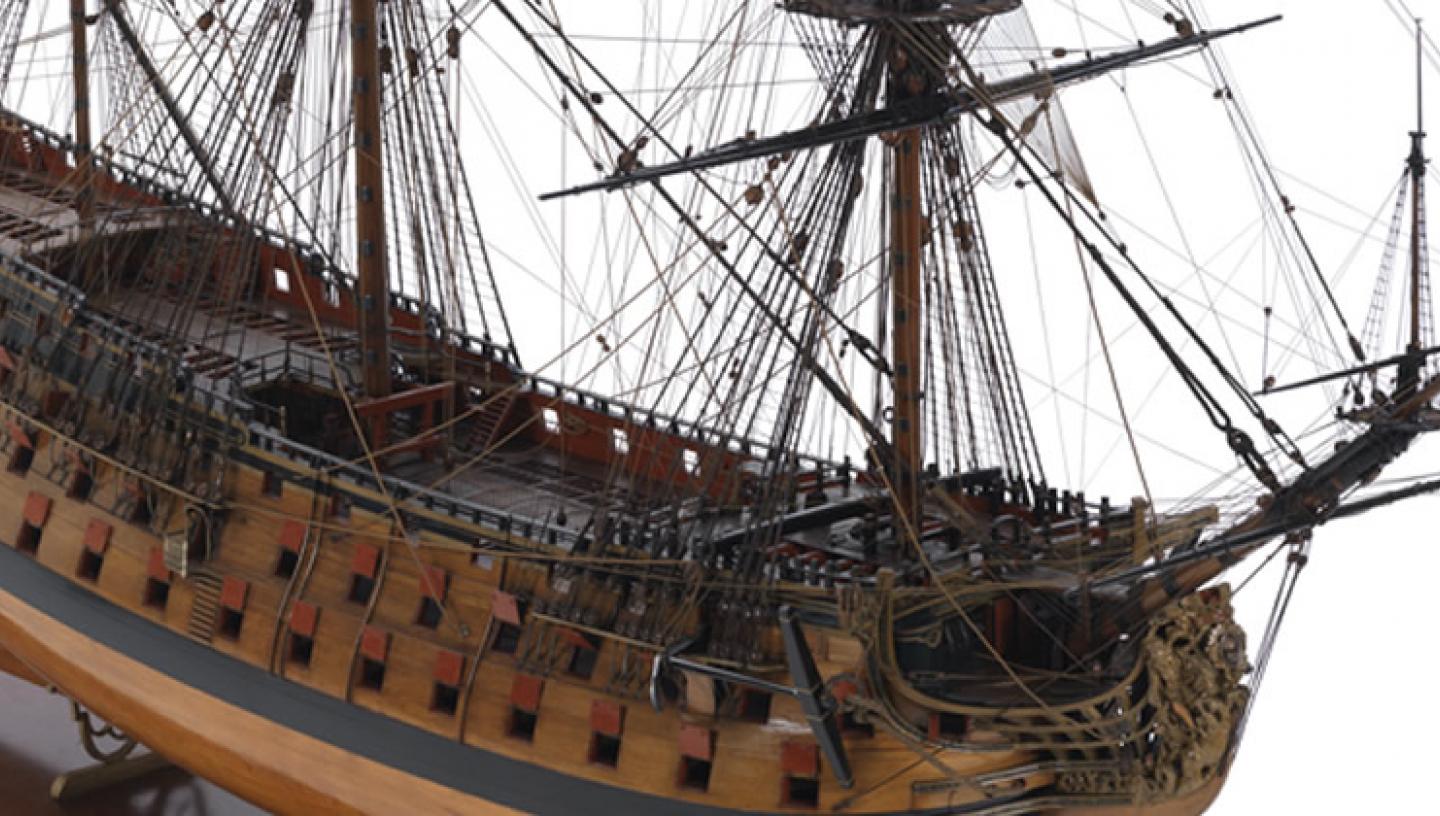This photograph showcases a detailed wooden model of an old sailing ship, reminiscent of the 17th or 18th century, similar to the era of the USS Constitution. The model is crafted from shiny polished wood and positioned on a display stand on a table, with only the lower left-hand corner of the table visible in the image. The ship features multiple wooden masts adorned with an extensive network of rigging and netting, attached to various points on the keel and extending from the top of the masts downwards. The deck of the ship is slightly darker brown than the medium brown sides. The bow of the ship boasts a metallic design, while the side of the ship is lined with more than a dozen cannon holes, or possibly windows, hinting at its multi-level structure. This rear-half view of the ship highlights its intricate assembly, with countless ropes or tiny strings stretching across the top and sides, emphasizing the ship's historical and maritime significance.